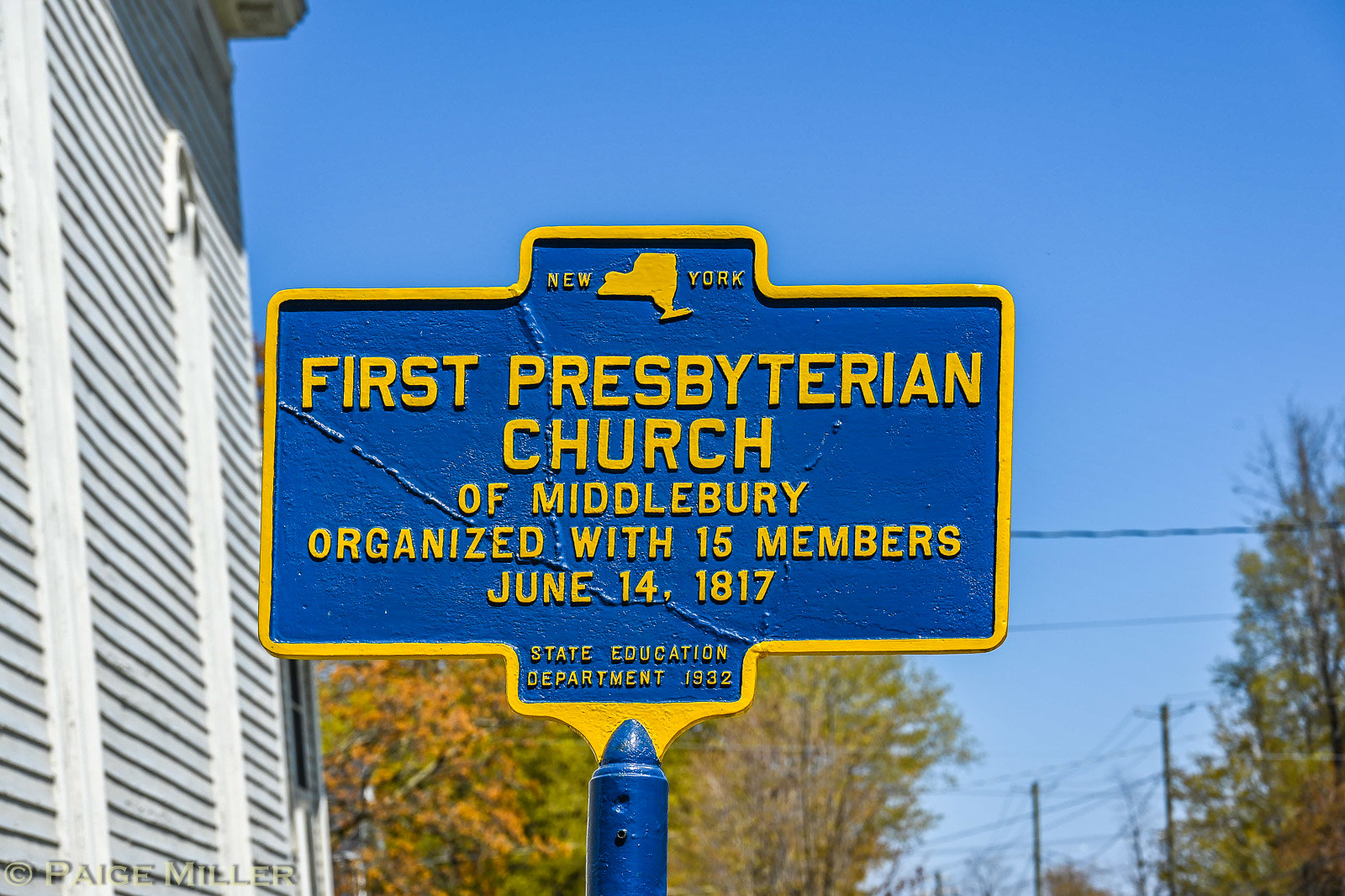In this picture, a vivid blue sky devoid of clouds serves as the backdrop, embracing both sides of the image with lush green trees that provide ample shade. On the far left, there stands a church with distinctive vertical wooden siding. The architectural detail includes a partial arch that suggests the presence of a window, though it is mostly obscured, hinting at either a design element or a partially visible window.

At the forefront of the image, a prominent blue sign with yellow text captures attention. The sign features a somewhat rectangular shape, embellished with two small rectangular protrusions at its top and bottom center. The sign reads "New York" at its summit, accompanied by a cut-out of the state's map in yellow. Beneath this, "First Presbyterian Church" is inscribed in large font over two centered lines, followed by "Of Middlebury" on the next line, and "Organized with 15 members" on the line below. Further down, it cites the date "June 14, 1817," and "State Education Department 1932" at the bottom. The sign has an elevated placement, which necessitates a view looking upward to fully observe its details.

Altogether, this image portrays a serene setting with historical significance, encapsulated in a crisp, sunny day framed by verdant foliage and a notable church landmark.